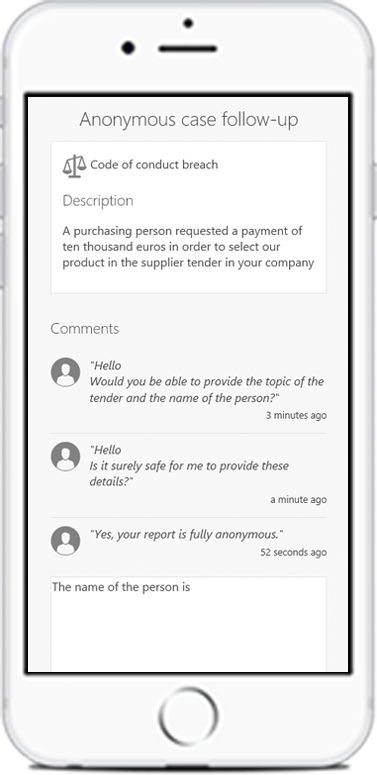The image depicts a detailed outline of a white cell phone, showcasing key features such as the back buttons on the left side and the volume buttons on both sides. At the top, there is a small black dot and a black line accompanied by another dot. The screen outline is highlighted in black.

The display shows a notification with a gray shaded background at the top, which reads "Anonymous Case Follow-Up." Below this, a white pop-up box contains text about the "Code of Conduct" with a small icon resembling attorney scales. The description reads: "A purchasing person requested a payment of 10,000 euros in order to select our product in the supplier tender in your company."

Following the description is a comments section, all in gray text. The first comment states: "Hello, would you be able to provide the topic of the tender and the name of the person?" This comment was posted three minutes ago and is separated from the next comments by fine lines. 

The subsequent comment asks: "Hello, is it surely safe for me to provide these details?" posted a minute ago. Another comment responds: "Yes, your report is fully anonymous," posted 52 seconds ago.

Underneath these exchanges is an additional white box, which seems to prompt the user to fill in the name of the person, though it remains blank. Each comment is accompanied by a gray circle featuring a white silhouette of a person, denoting user icons.